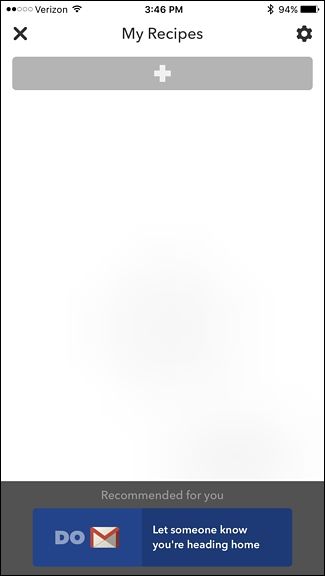The image appears to be a screenshot of a smartphone screen. In the upper left corner, the word "Verizon" indicates the cellular provider, accompanied by a Wi-Fi symbol. Positioned at the top center is the current time, displayed as 3:48 p.m. On the top right corner, a battery icon is visible.

Beneath the time display, centered at the top of the screen, the text "My Recipes" is prominently shown. Just below this, a large gray box stretches across the width of the screen, featuring a white plus sign in its center, likely serving as a button to add new content.

The main portion of the screen is predominantly blank and white, indicating an empty state, suggesting that no recipes have been added yet.

At the very bottom of the screen, there is a gray box labeled "Recommended for you." Inside this box, a smaller blue rectangle contains the text "Do," accompanied by an envelope icon in red and white, and a message that reads, "Let someone know you're heading home."

Overall, the page seems to be designed for users to enter and manage recipes, but it is currently in an empty state with no recipes added.